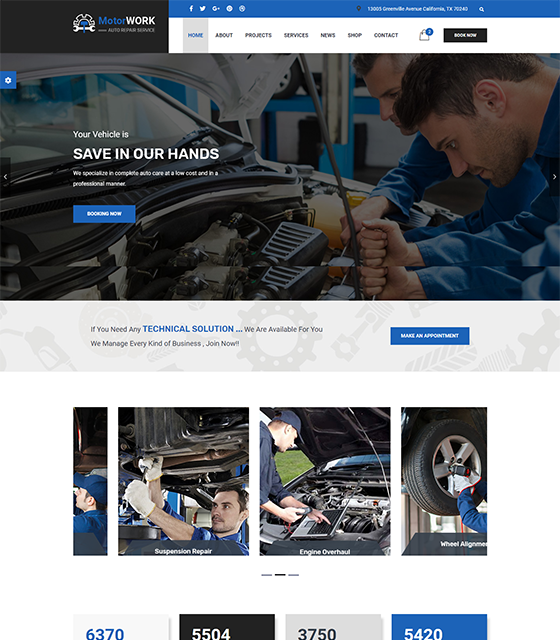**Homepage Screenshot of Motor Work Auto Repair Service Website**

At the top of the homepage, there are three main headers. 

1. On the top left, a dark gray header displays the brand's name: "Motor Work", with "Motor" in blue and "Work" in white, followed by "Auto Repair Service". A white wrench icon serves as the logo to the left of this text.
 
2. To the right, a smaller, blue header runs across the top of the screen. This section contains social media logos on the top left. On the top right, it displays the address: "13093 Greenville Avenue, California, Texas 79240". A white magnifying glass icon is located to the right of the address.

3. Beneath the blue header, a white navigation bar provides several options. The "Home" option is highlighted in light gray with blue text, while the remaining options—"About," "Projects," "Services," "News," "Shop," and "Contact"—are in dark gray. A shopping bag icon with a blue circle and a white number two is next to the "Contact" option. To its right, there is a black button labeled "Book Now" in white text.

Beneath the headers, a darkened image depicts two men working on a car engine. Both men have short brown hair and are wearing blue shirts. Overlaying this image, white text states: "Your vehicle is safe in our hands. We specialize in complete auto care at a low cost and in a professional manner." Beneath this is a blue button with white text that reads "Book Now."

Following the image, a gray background features various icons such as cogs and gas pumps. The section includes text in blue: "If you need any technical solution, we are available for you. We manage every kind of business. Join now!!" To the right, a blue button with white text invites users to "Make an Appointment".